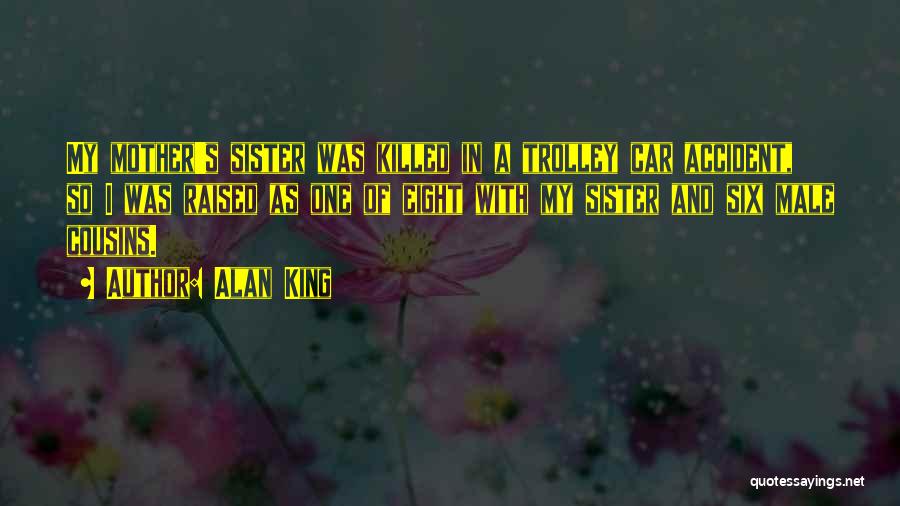The image features a quote by author Alan King, presented in a unique style where the yellow lettering juxtaposes transparency revealing the dim, dark background. The text reads, "My mother's sister was killed in a trolley car accident, so I was raised as one of eight with my sister and six male cousins." The quote is in uppercase gray text, set inside yellow bars, forming the most prominent element against the gloomy backdrop. The background itself displays an out-of-focus image of purple flowers with yellow centers and thin green stems, shrouded by raindrops and augmented by an overall dark, subdued, and near opaque blue-green-gray hue. The image carries a melancholic, dreary tone, emphasizing the somber content of the quote. At the bottom right corner is the text “quotesayings.net” in small white letters.